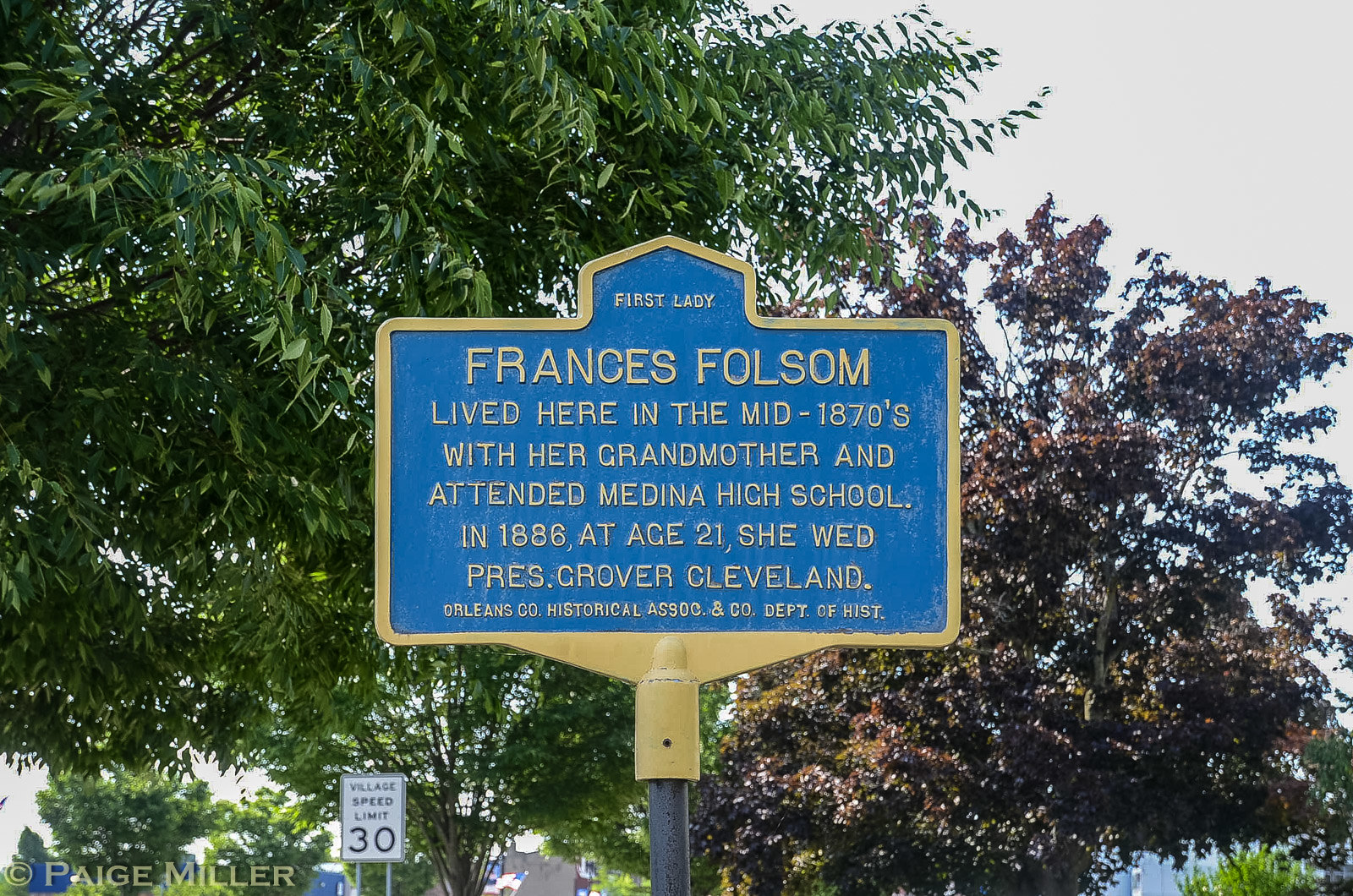This horizontally oriented photograph captures an idyllic outdoor scene dominated by trees and an informational sign. The background features a mix of sky and foliage, with the upper right-hand corner showing a grayish-blue sky. The left side of the image is framed by a tree with vibrant green leaves, while the right side showcases a tree adorned with purplish leaves.

Centrally positioned on a single metal pole is a prominently featured historical sign. The sign is rectangular with a gold border and a blue background, embellished with gold text. At the very top, it reads "First Lady," followed by "FRANCES FOLSOM" in large, all-caps letters. The text below in slightly smaller all-caps letters details that she lived in the area in the mid-1870s with her grandmother and attended Medina High School. It further notes that in 1886, at age 21, she married President Grover Cleveland. At the bottom of the sign, in smaller print, it states, "Orleans County Historical Association and Company Department of History." The sign also features a peaked roof structure.

In the lower left corner of the photograph, there is a speed limit sign displaying "Village Speed Limit 30," and nearby, the name "Paige Miller" appears with a copyright symbol. Complimenting the scene, the overall lighting suggests a bright but overcast day, enhancing the natural hues of the trees and the crisp details of the sign.